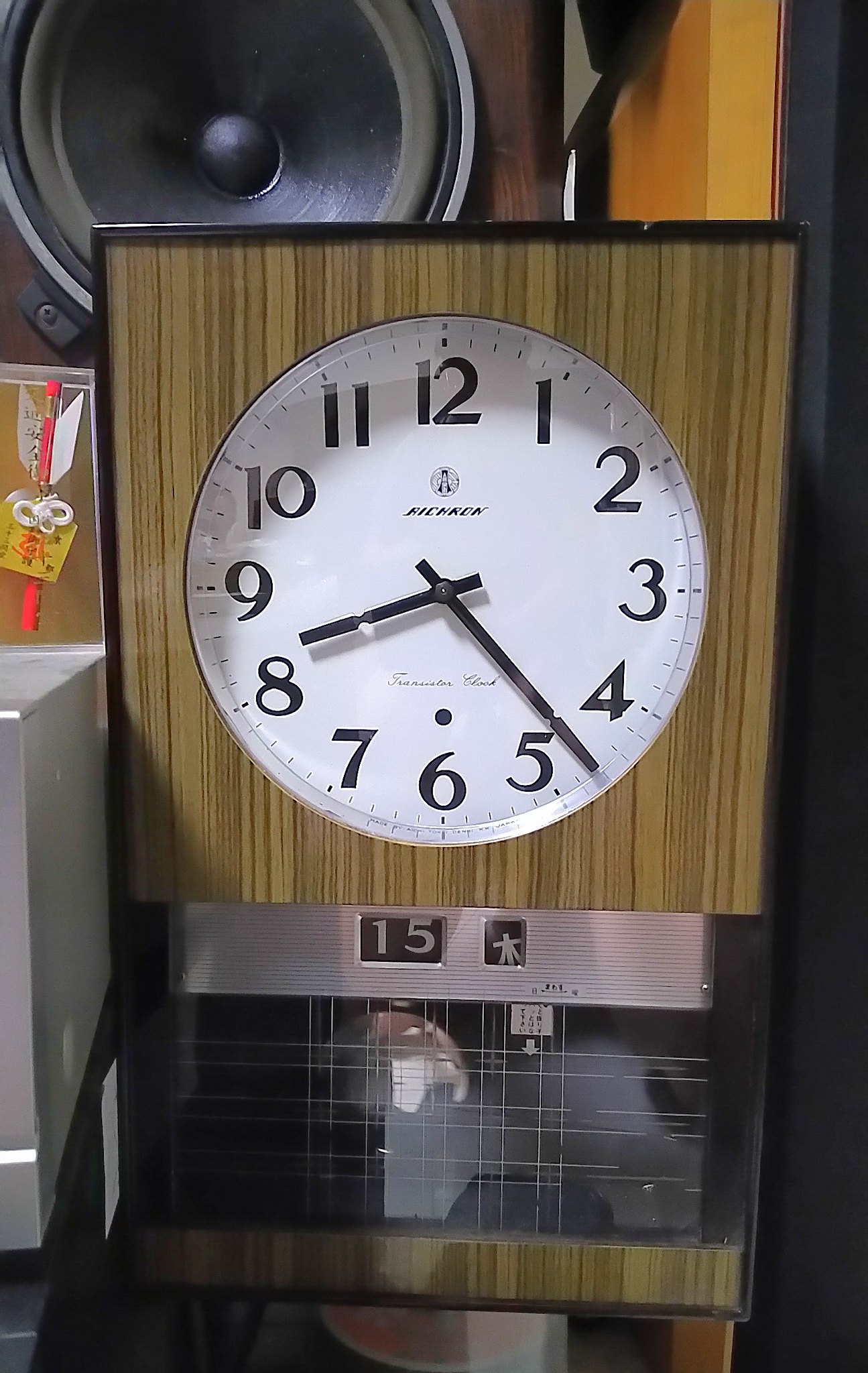In this portrait-oriented photograph, the centerpiece is a rectangular wall clock occupying the majority of the frame. The clock's upper two-thirds feature a pristine white face adorned with bold black numerals and matching black minute and hour hands, indicating the time as 8:23. Enveloping the clock face is a sophisticated wood grain pattern that adds a touch of warmth and texture to the timepiece.

Behind the clock, partially visible, is the lower section of a sleek black audio speaker encased in a darker wood finish, providing a contrast to the lighter tones of the clock. To the left of the main scene, a pencil rests on an unidentified object, subtly hinting at an organized and productive setting.

Beneath the clock face, the number '15' is prominently displayed in a black square, possibly indicating a date or part of a larger mechanism. Below this numerical display, a metallic pattern can be seen, adding an element of industrial design to the composition. The rest of the background remains plain, allowing these details to stand out prominently.